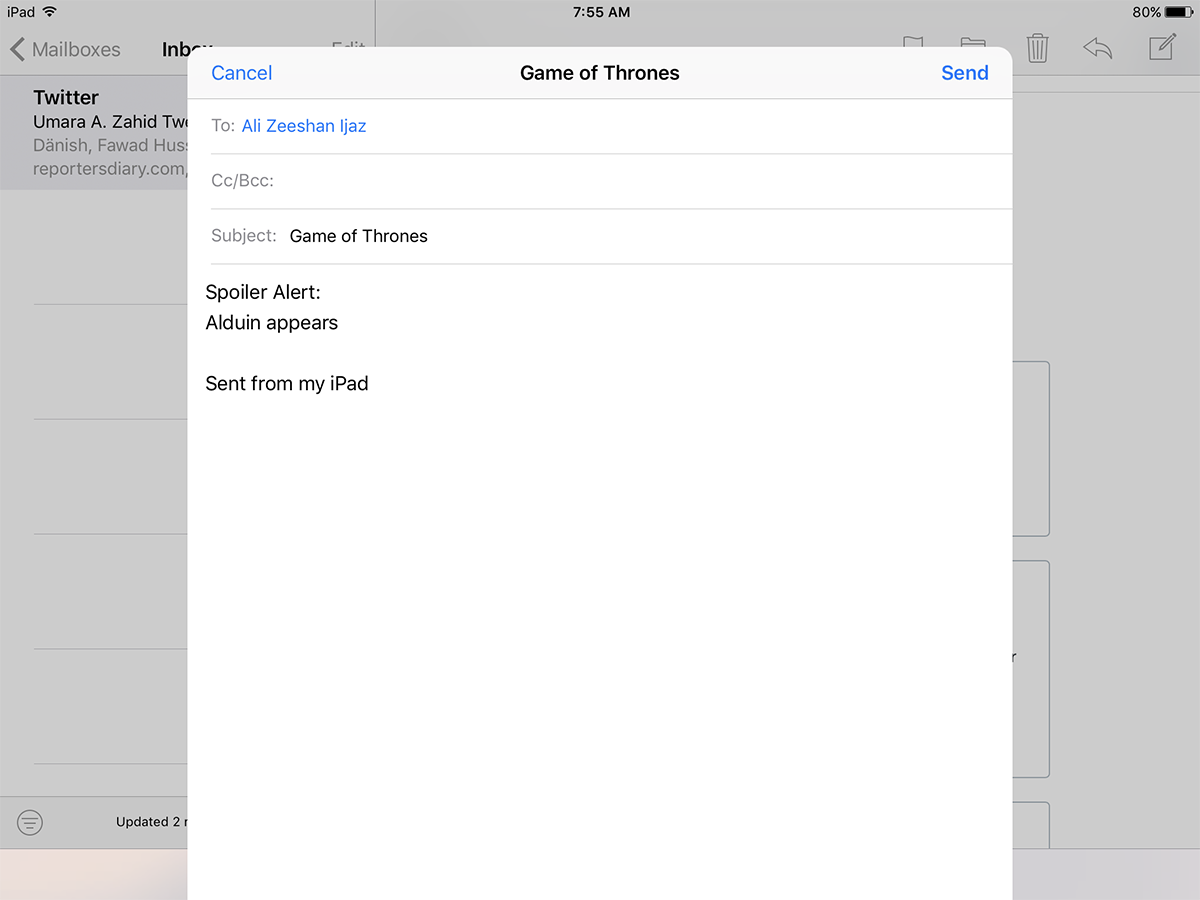The image depicts an iPad screen displaying a pop-up message overlaying a Mail application. The Mail app interface shows a gray background with "Mailboxes" and "Inbox" partially visible behind the pop-up. The pop-up itself has a white background and is in the process of composing an email. 

The composition fields of the email are as follows:
- **To**: Ali Z. Shan, with the email address zeshanljaz@example.com.
- **Subject**: Game of Thrones (Spoiler Alert: Alduin appears).

At the bottom, there is a line indicating the email was "Sent from my iPad."

The pop-up message presents two options: "Cancel" on the left and "Send" on the right, both in blue text. The status bar at the top of the iPad screen shows it is 7:55 a.m., the Wi-Fi connection is active, and the battery is at 80% charge.

This moment captures the user actively working on an email draft, containing spoilers about "Game of Thrones," but it has not yet been sent or canceled.